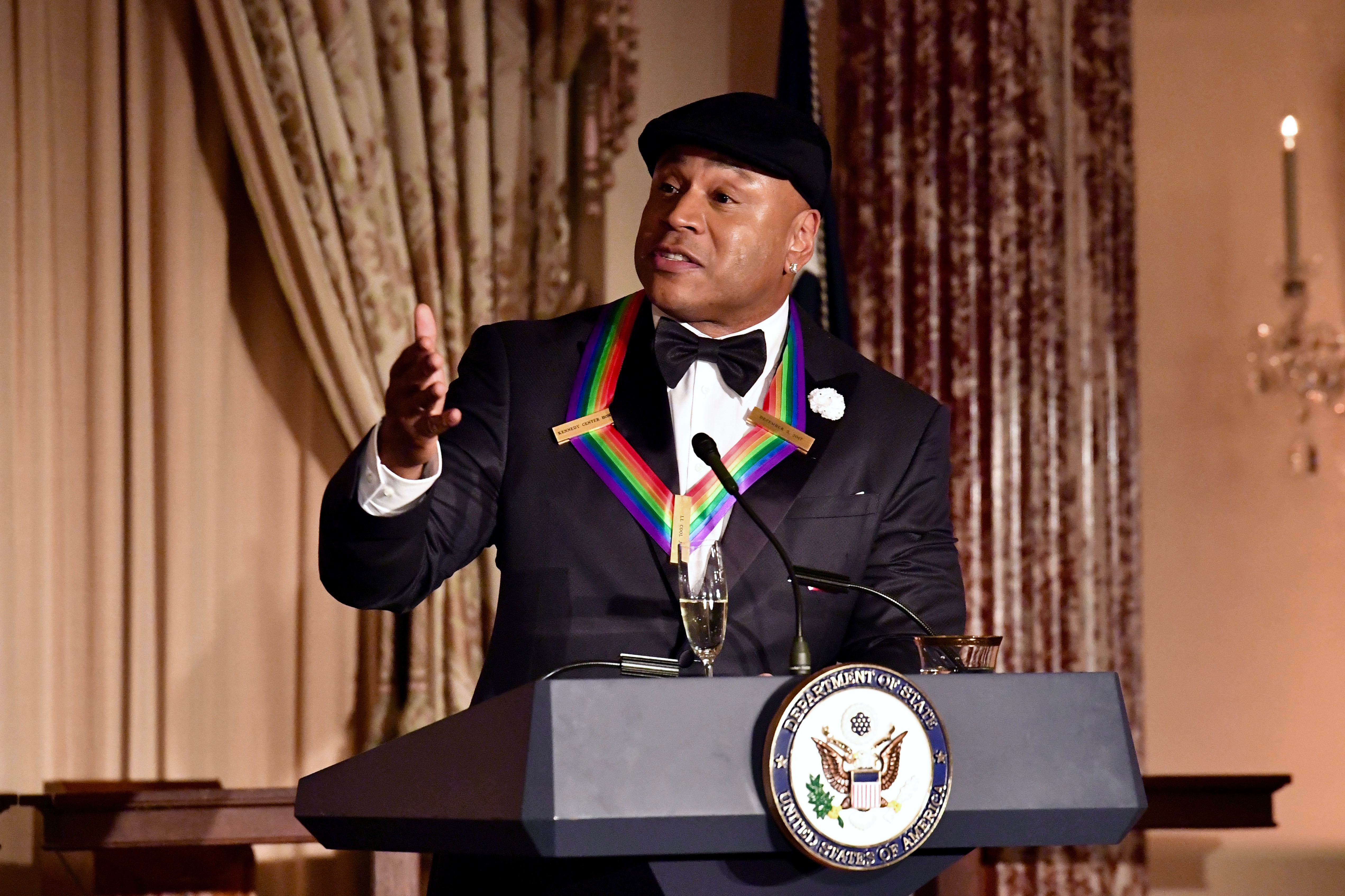In the image, LL Cool J stands at a black podium adorned with the presidential seal, which is white with blue accents and features the American Eagle, reading "Department of State, United States of America." Behind him hang elegant light brown curtains, and candelabras are affixed to the walls, enhancing the room's opulent atmosphere. LL Cool J, donning a dark cap, is impeccably dressed in a black tuxedo with a white undershirt and a black bow tie. His outfit is complemented by a notable rainbow-colored ribbon around his neck, featuring shades from red to green to blue to purple. A small white flower decorates his lapel. Positioned next to a microphone on the podium is a half-full champagne glass. LL Cool J is caught in a gesture with his right hand extended forward, and he is looking off to the left.